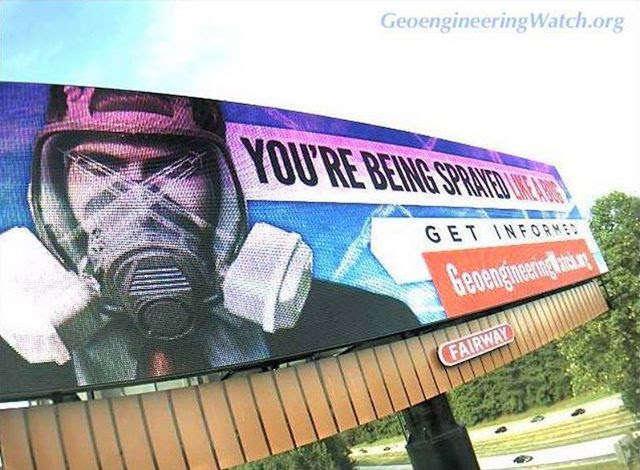The photograph captures a colorful billboard during daytime. The central illustration features a man donning a sophisticated face mask equipped with white ventilators on either side, a large, clear white visor, and a dark-colored grill with vents covering his mouth. The mask is secured with straps around his head, and the man has dark, straight hair.

Adjacent to this illustration, a bold banner reads, "YOU'RE BEING SPRAYED LIKE A DOG." Below that, on a white banner, the slogan "GET INFORMED" is prominently displayed, followed by another banner in red that states "GEOENGINEERINGWATCH.ORG." The background of the billboard showcases a blue sky crisscrossed with lines.

In the distance, the scene includes green foliage from trees, roadways bustling with traffic moving in two directions, and a blue sky dotted with fluffy white clouds. The top corner of the image is stamped with the website "GEOENGINEERINGWATCH.ORG," linking back to the billboard's message.